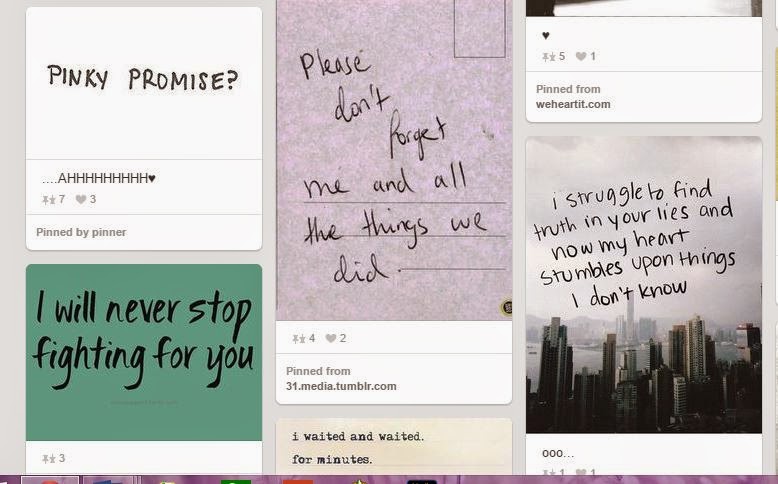The image is a collage divided into three columns, each containing partial rectangles or squares featuring clips of various posts.

- **First Column:** 
  - The top section displays the phrase "Pinky Promise?" followed by a horizontal line, the exclamation "A H H H H H H," and a black heart icon. Below this, there's an indicator for a pinned post with "pinned by pinner," accompanied by a "pin down" and "pin up" icon, a number '7,' and a heart with the number '3.' 
  - The next segment has a green background with the text, "I will never stop fighting for you." Similar to the previous, there's a "pin up" and "pin down" icon alongside the number '3.'

- **Second Column:** 
  - The upper part features text on a gradient background blending pink and gray hues. It reads, "Please don't forget me and all the things we did," resembling a postcard. This section includes a "pin down" and a "pin up" icon with the number '4,' a heart with the number '2,' and the note "pinned from 31.media.tumblr.com."
  - Below, there is off-white text reading, "I waited and waited for minutes," with an obscured image in the upper right corner. This part of the column includes a heart icon, "pin down" and "pin up" signs with the number '5,' a heart with the number '1,' and "pinned from weheartit.com."

Each column presents a unique blend of messages, hearts, and pin indicators, creating an intricate and colorful tapestry of emotional quotes and digital interactions.